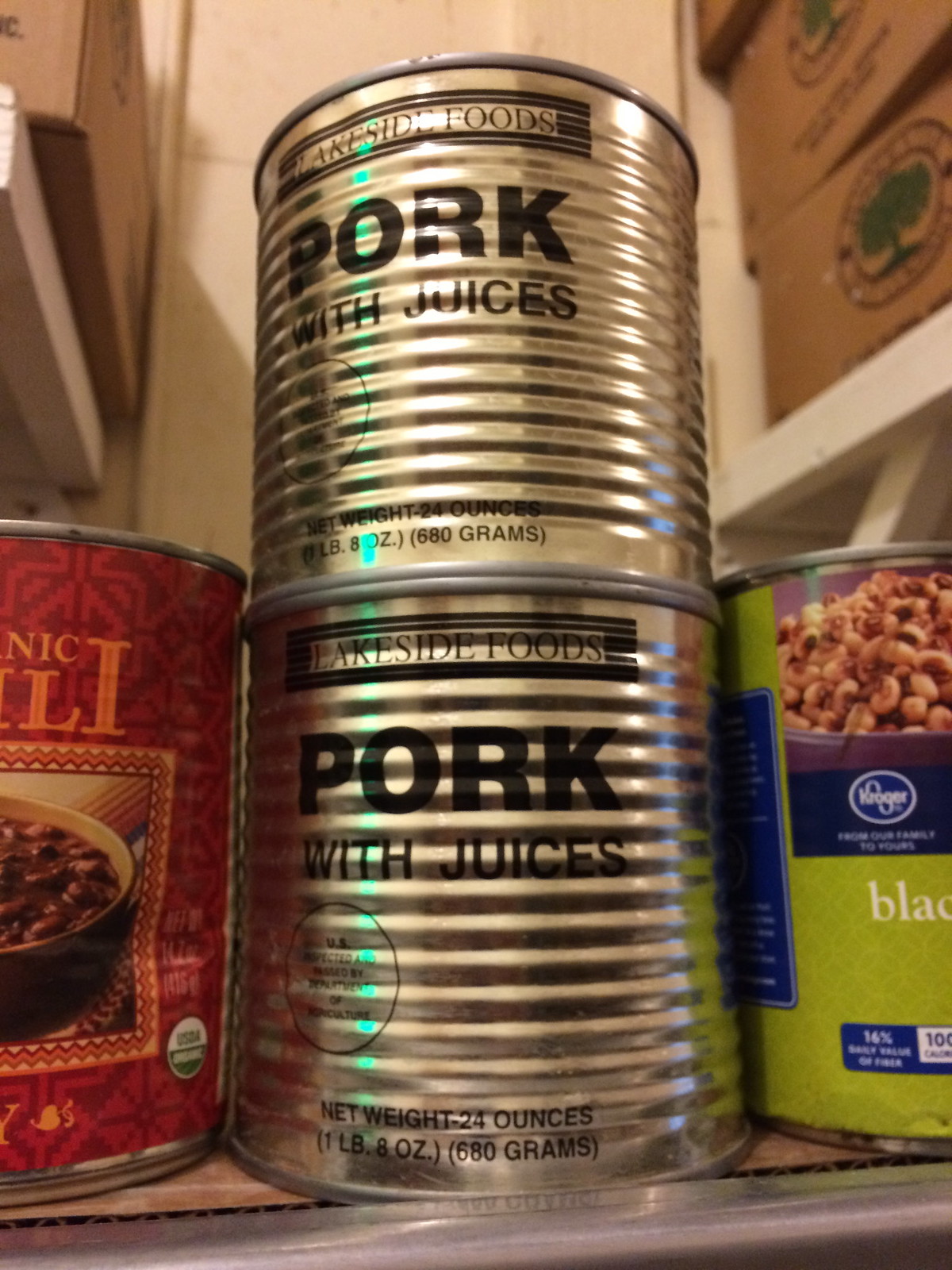This indoor color photograph captures a detailed scene, likely from a pantry or grocery store shelf. The focal point of the image features two tin cans stacked neatly atop each other on a brown cardboard surface. These cans are silver, horizontally ribbed, and bear the printed label "Lakeside Foods" in large black capital letters, followed by "Pork with Juices." A USDA inspection stamp is visible in a circle on the bottom left of the cans. Below, the label states "Net Weight 24 ounces" (1 lb. 8 oz. / 680 grams). Flanking the central cans, partially off-screen, are two additional cans; one appears to have a red label indicating chili, while the other has a green label showing a bowl of beans. In the upper right corner, a stack of boxes is visible, and in the upper left, another box sits on a shelf. A silver steel pole extends horizontally in front of the cans, suggesting the presence of shelving or a countertop edge. The background reveals a white wall, adding context to the pantry-like setting.